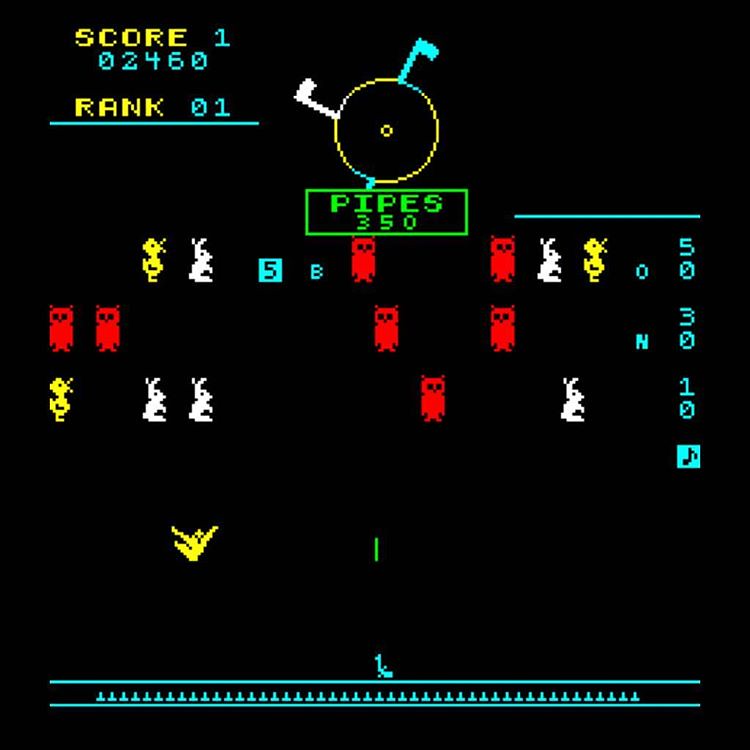This image depicts a screen from a retro 8-bit video game set against a black background. Prominently displayed at the top left in yellow is the label "SCORE" followed by the number "1" in teal, with the score "02460" in teal just below it. The word "RANK" is shown in yellow, accompanied by "01" in teal, which sits above a teal horizontal bar. In the upper center, there's a stylized yellow circle adorned with two flags—one teal, one white. The bottom of the screen features a green-outlined rectangle labeled "PIPES," containing the number "350" in green text. Various 8-bit animals populate the screen, including red owls, white bunnies, and yellow ducks. Near the bottom, a yellow bird appears to be in flight. Below the bird, two teal lines run horizontally with arrow-like figures pointing upwards, resembling the barrels of a dual-shooter game. This pixelated scene clearly illustrates an old-school shooting video game environment.